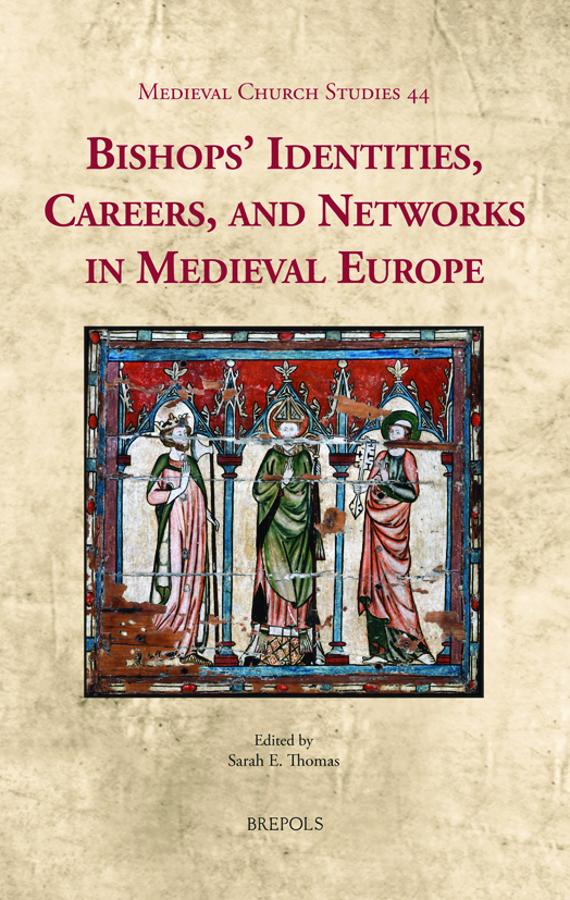The image depicts the cover of a book titled "Medieval Church Studies 44: Bishops, Identities, Careers, and Networks in Medieval Europe." The book cover, which has an aged, pinkish-beige tone with a marbled pattern, features a detailed depiction of three medieval bishops in different costumes, set against a white background. Each bishop is dressed in long gowns, with the one on the right wearing a green halo, the middle one with an orange halo, and the left one wearing a crown. The backdrop of the image includes blue pillars and arches, giving a sense of historical church iconography. The cover text, written in red at the top, is followed by the names of the editor, Sarah E. Thomas, and the publisher, Brepols, printed in black text at the bottom of the cover.